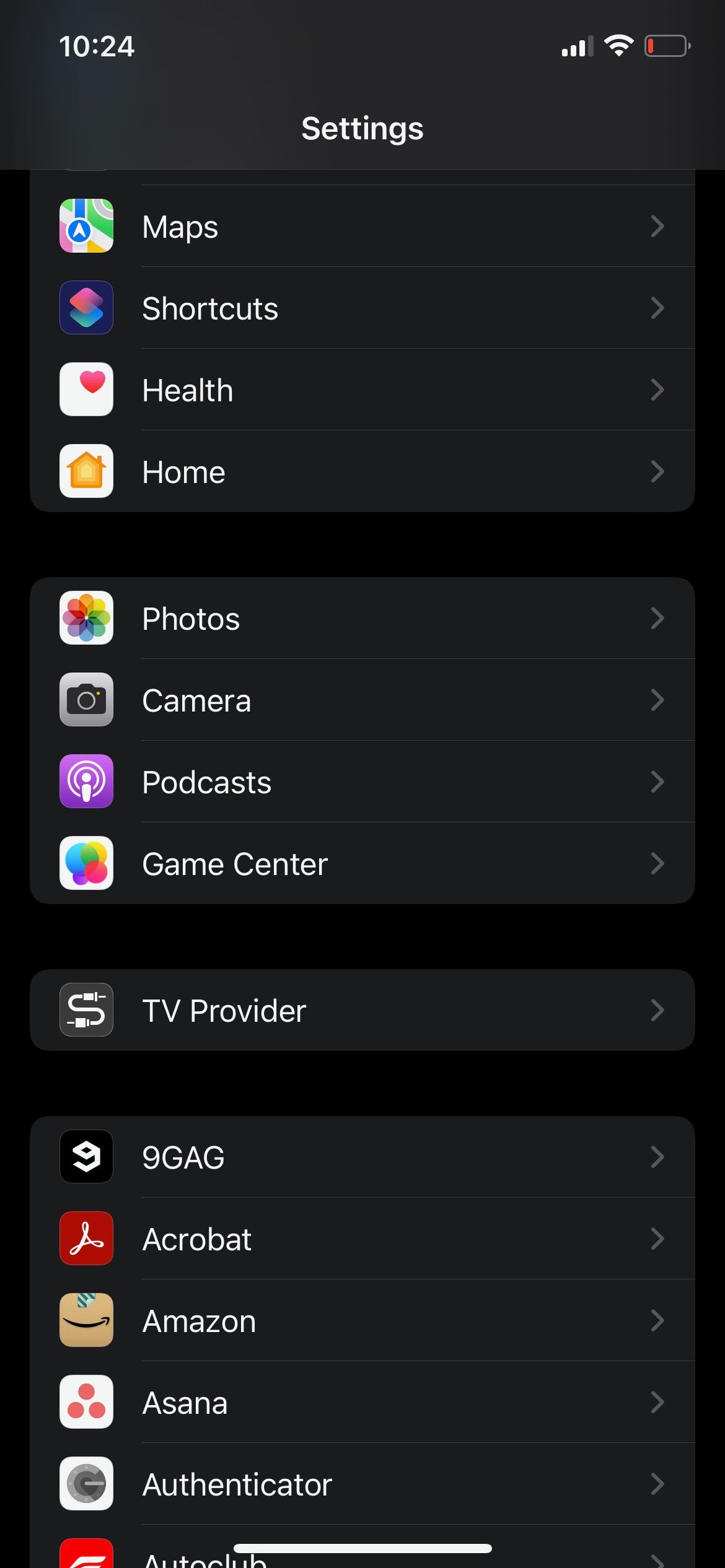This screenshot from a cell phone displays a dark matte black background with a header at the top. The time, "10:24," is displayed prominently in white on the top left corner. To the right, the screen indicates strong connectivity with three out of four bars, shows active Wi-Fi, and depicts a nearly depleted battery with the icon in red.

Centered on the screen is the title "Settings" in white, followed by a comprehensive list of navigation options. Each option is paired with an icon on the left and the name on the right. The icons are detailed and color-coded for easy identification:

1. **Maps**: Accompanied by a map logo.
2. **Shortcuts**: Displayed with a shortcut icon.
3. **Health**: Represented with a white square containing a heart.
4. **Home**: Illustrated with a white square featuring a house.
5. **Photos**: Depicted with a white square adorned with a flower.
6. **Camera**: Shown with a gray square housing a camera icon.
7. **Podcasts**: Marked by a blue square with a microphone.
8. **Game Center**: Identified by a white square with multicolored circles.

Following this set, there is another grouping of applications:

9. **TV Provider**: Indicated by a black square with connected wires.
10. **9GAG**
11. **Acrobat**
12. **Amazon**
13. **Asana**
14. **Authenticator**
15. **Autoclub**

The list continues but the text is cut off at this point.